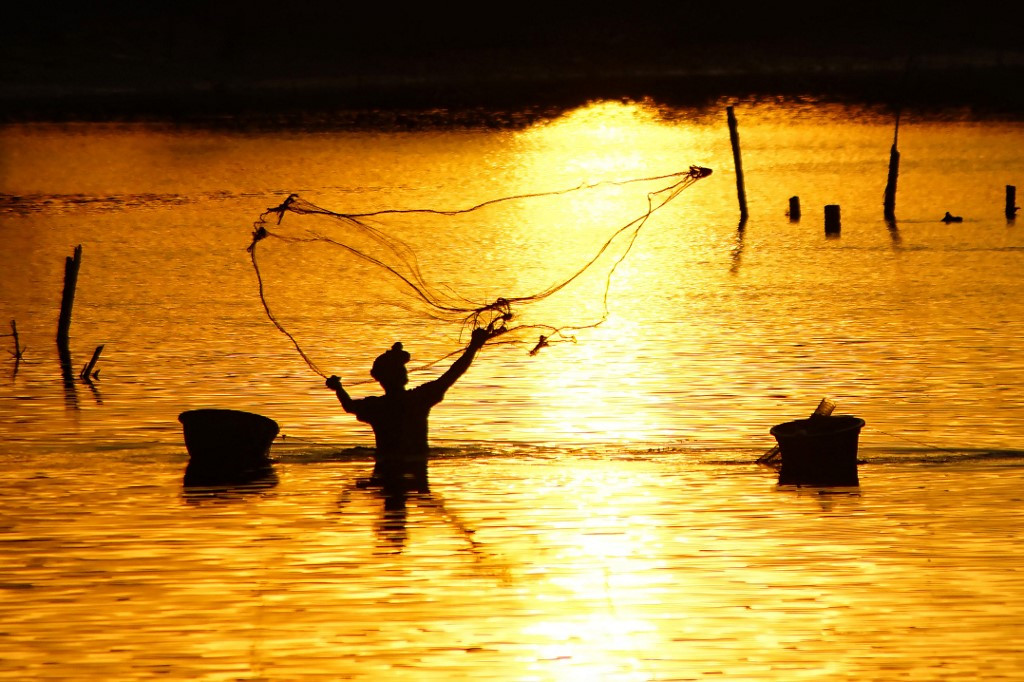In this striking silhouette image, a person stands waist-deep in a vast, shimmering body of water—possibly an ocean or lake—casting a fishing net at sundown. The tranquil water, illuminated by the golden hues of the setting sun, enhances the scene's serene beauty. The angler, positioned slightly to the left of the central frame, has just thrown the net, which is gracefully suspended mid-air. Surrounding them are numerous items: two large buckets floating nearby, one on each side, and several poles and branches jutting out of the water, adding depth and texture to the composition. In the background, the vivid colors of the sunset—yellows, oranges, and light oranges—blend seamlessly, creating a picturesque and peaceful atmosphere.